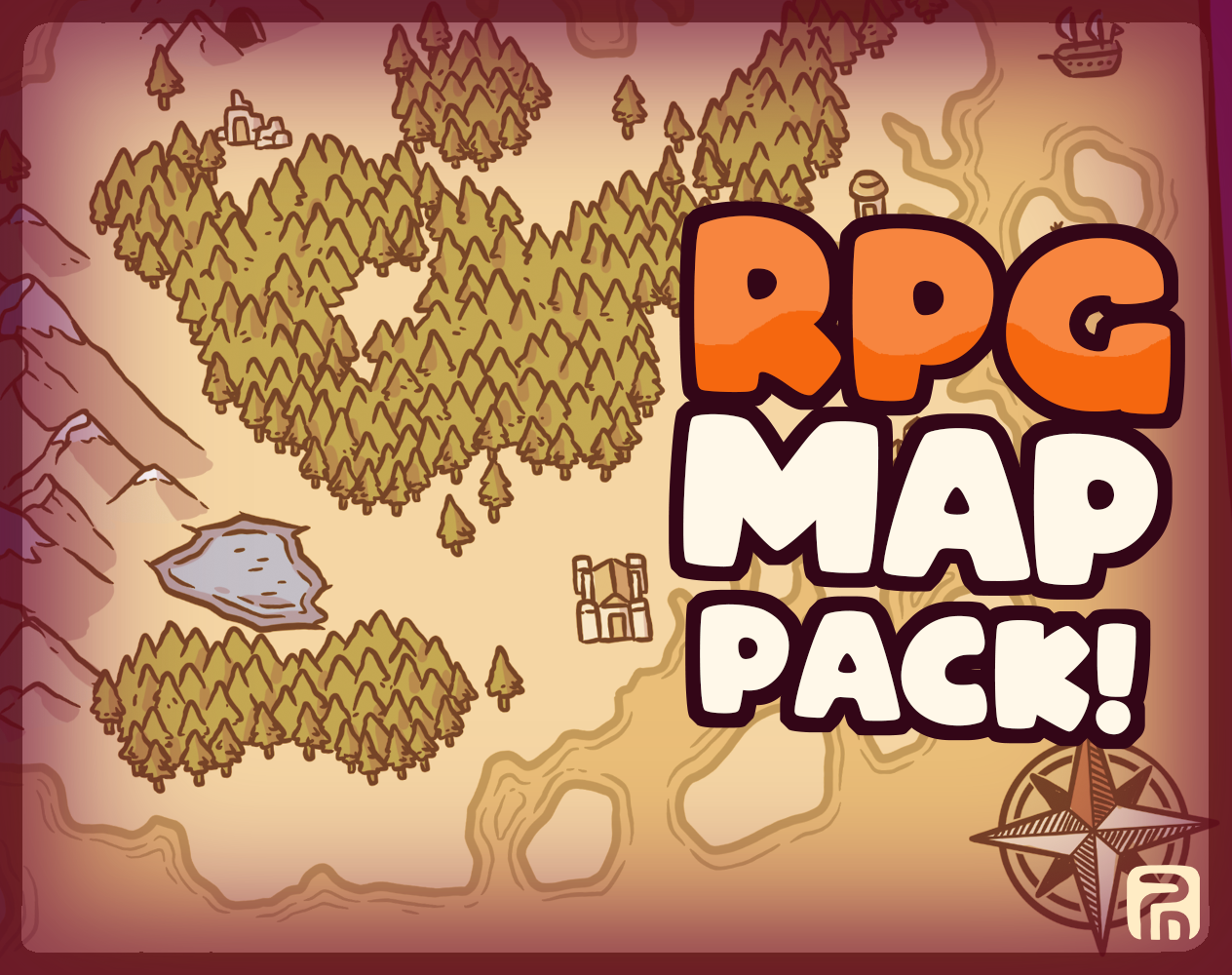The image features a color illustration in landscape orientation, serving as a map pack cover for a role-playing game (RPG). The background boasts a pinkish and tan gradient, with the words "RPG" in bold orange gradient, and "map pack!" in white letters with a black outline, prominently displayed on the right. The map itself is simplistic yet detailed, depicting a large, forested landscape with hundreds of green trees clustered together. To the west, there are mountain cliffs, with a small lake nestled at their base. The map also showcases various other topographic features, such as a small building in the center, a two-masted sailing ship near the top right, suggesting the proximity of an ocean or large body of water, and some small islands off the coast. Additionally, a compass rose symbol decorates the lower right corner, likely indicating the Cardinal Ordinance or manufacturer's marker. The style seamlessly blends color illustration with graphic design and typography, presenting an inviting preview of the maps contained within the RPG map pack.